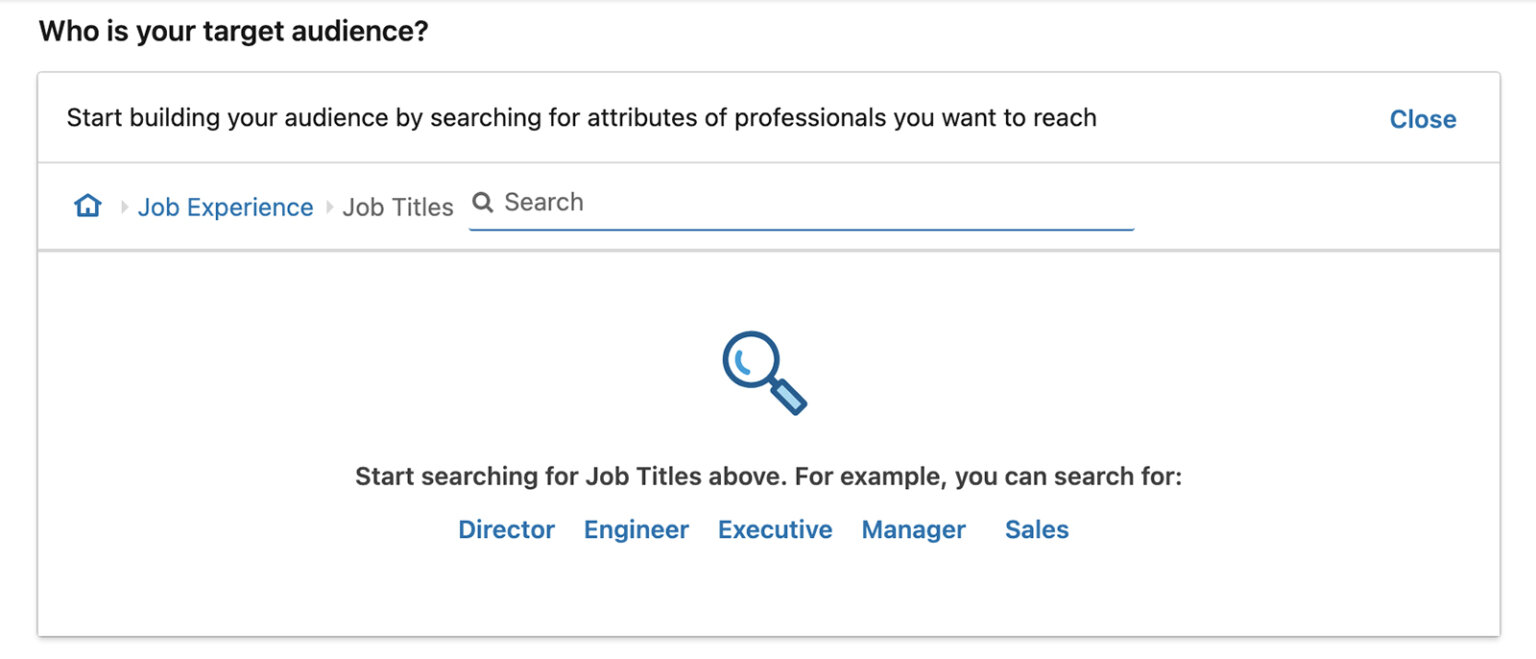**Detailed Caption:**

The image showcases a user interface of a website or application designed for audience targeting and search functionalities. The overall background is predominantly white, offering a clean and uncluttered visual. Positioned at the top left-hand side in bold lettering, it reads, "Who is your target audience?" Framing the primary content, a subtle grey box encompasses the remainder of the screen, providing a distinct separation from the white backdrop.

At the top center, a black text prompt states, "Start building your audience by searching for attributes of professionals you want to reach." Adjacent to this text on the right-hand side, the word "Close" is highlighted in blue, indicating an option to dismiss the menu.

Beneath this section, there is a small blue icon resembling a house, typically denoting a 'Home' function. Alongside the house icon, also in blue, is the text "Job Experience." Following this, another search criterion labeled "Job Titles" appears, accompanied by a grey magnifying glass icon that bears the word "Search," signifying the search action.

A prominent blue line runs horizontally across the interface, demarcating the search bar from further instructional content. Below this divider, a larger magnifying glass icon is displayed, with an instructional message reading: "Start searching for job titles above." The text then provides examples of potential search keywords in blue, such as "Director," "Engineer," "Executive," "Manager," and "Sales."

This detailed overview encapsulates the visual and functional elements presented in the application or website interface, highlighting key features and interactive components.